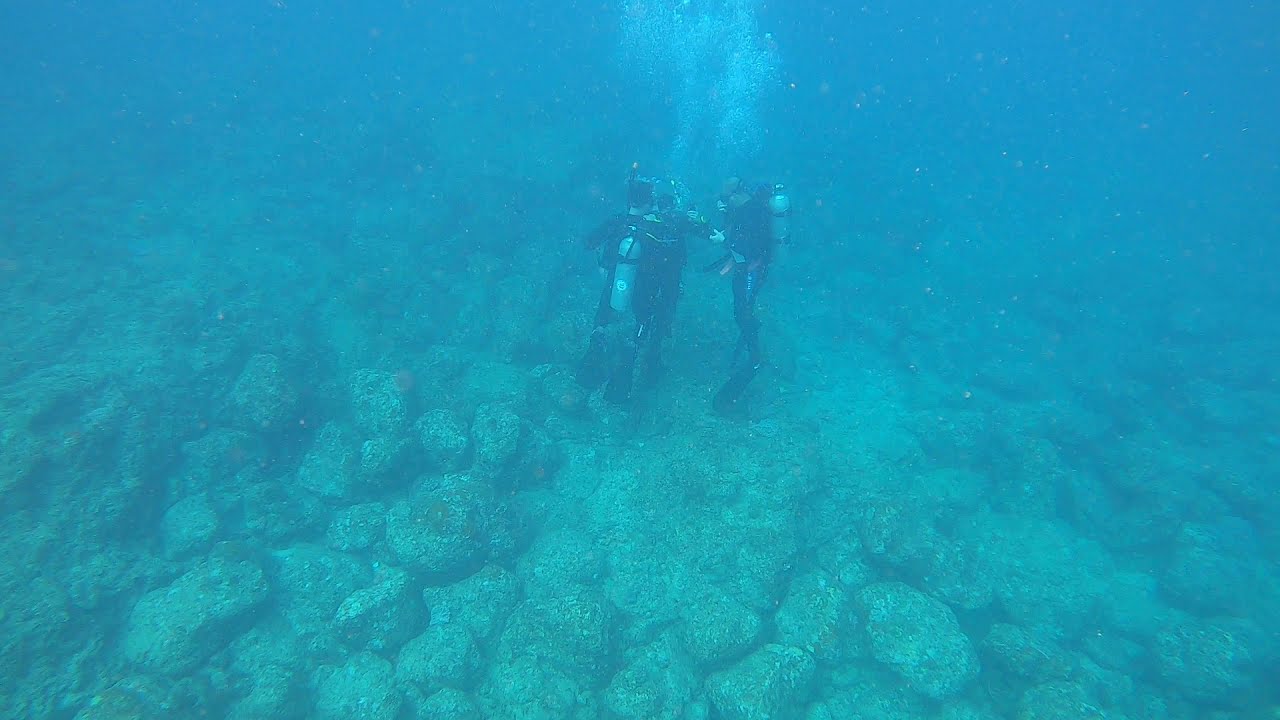This underwater photograph captures a vibrant blue scene, likely from a Mediterranean ocean, with slightly murky water that provides decent visibility up to 20 feet. The marine floor is dominated by an expanse of large, rocky boulders, some measuring several feet in size. These rocks appear to be covered with barnacles or small coral formations. The focus of the image is on three scuba divers positioned centrally. They are equipped with single tanks on their backs, and flippers on their feet, with air bubbles rising from their breathing apparatuses. The divers are seen at varying angles—one with his back to the viewer and the other two viewed from the side. This dynamic underwater scene is bathed in a light blue hue, reinforcing the sense of depth and the aquatic environment.